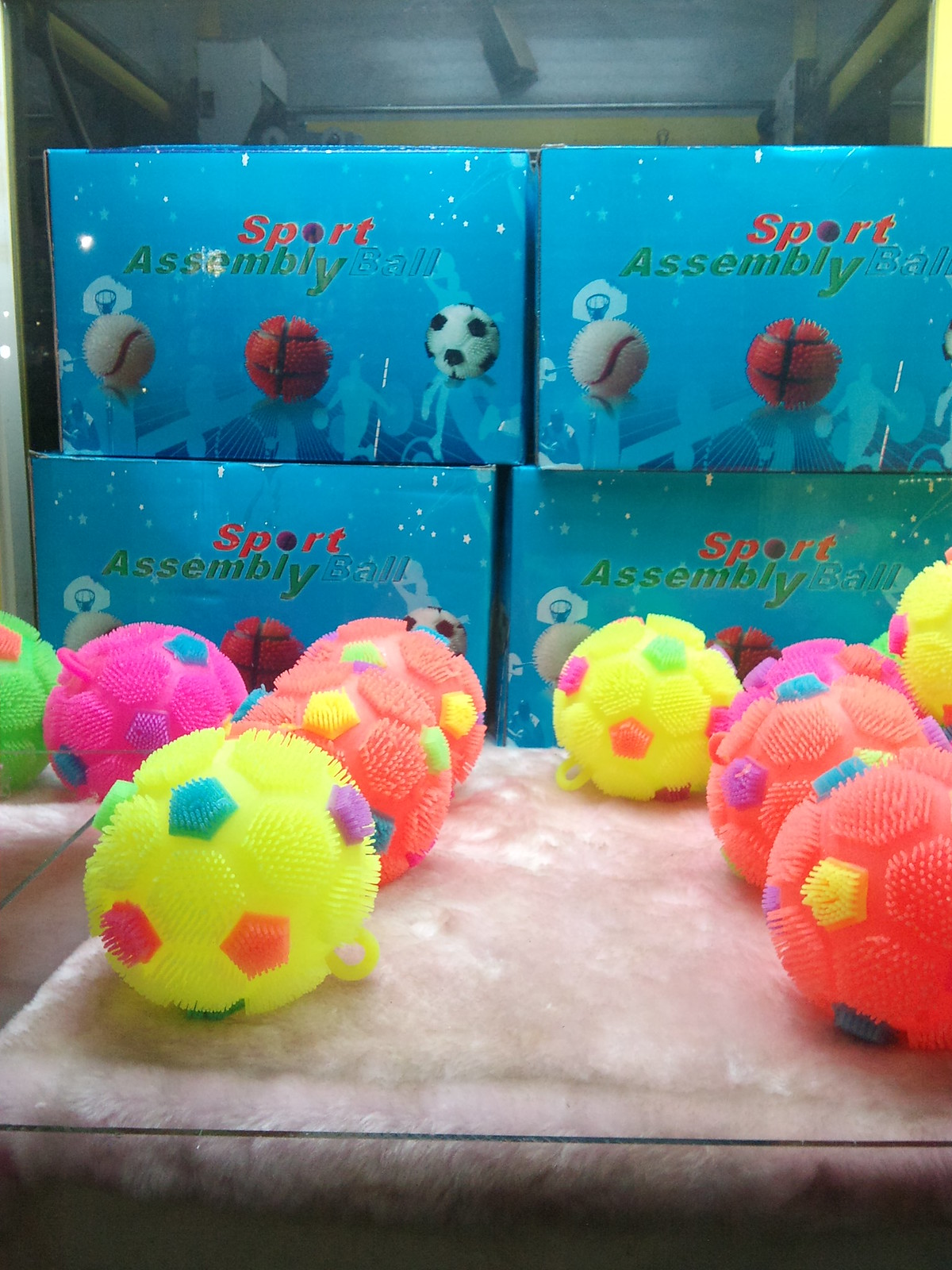The image features a collection of small, multi-colored rubber balls that resemble a combination of chew toys and sports balls, displayed on a shaggy cream or white rug under a glass container. The balls, which come in vibrant colors such as yellow, tangerine, peach, green, and pink, are covered in rubber filaments or tentacles that give them a squishy texture and enhance grip. Each ball is adorned with colorful dots of varying shades, including blues, reds, oranges, purples, and greens. These details make them appear playful and tactile. Behind the balls, there are blue boxes labeled "Sport Assembly Ball." The text on the boxes features "Sport" in red, using a purple ball as the "O," "Assembly" in green, and "Ball" in blue. The boxes display images of different sports balls—baseball, basketball, and soccer ball—and silhouettes of people engaged in active play, enhancing the sporty theme.